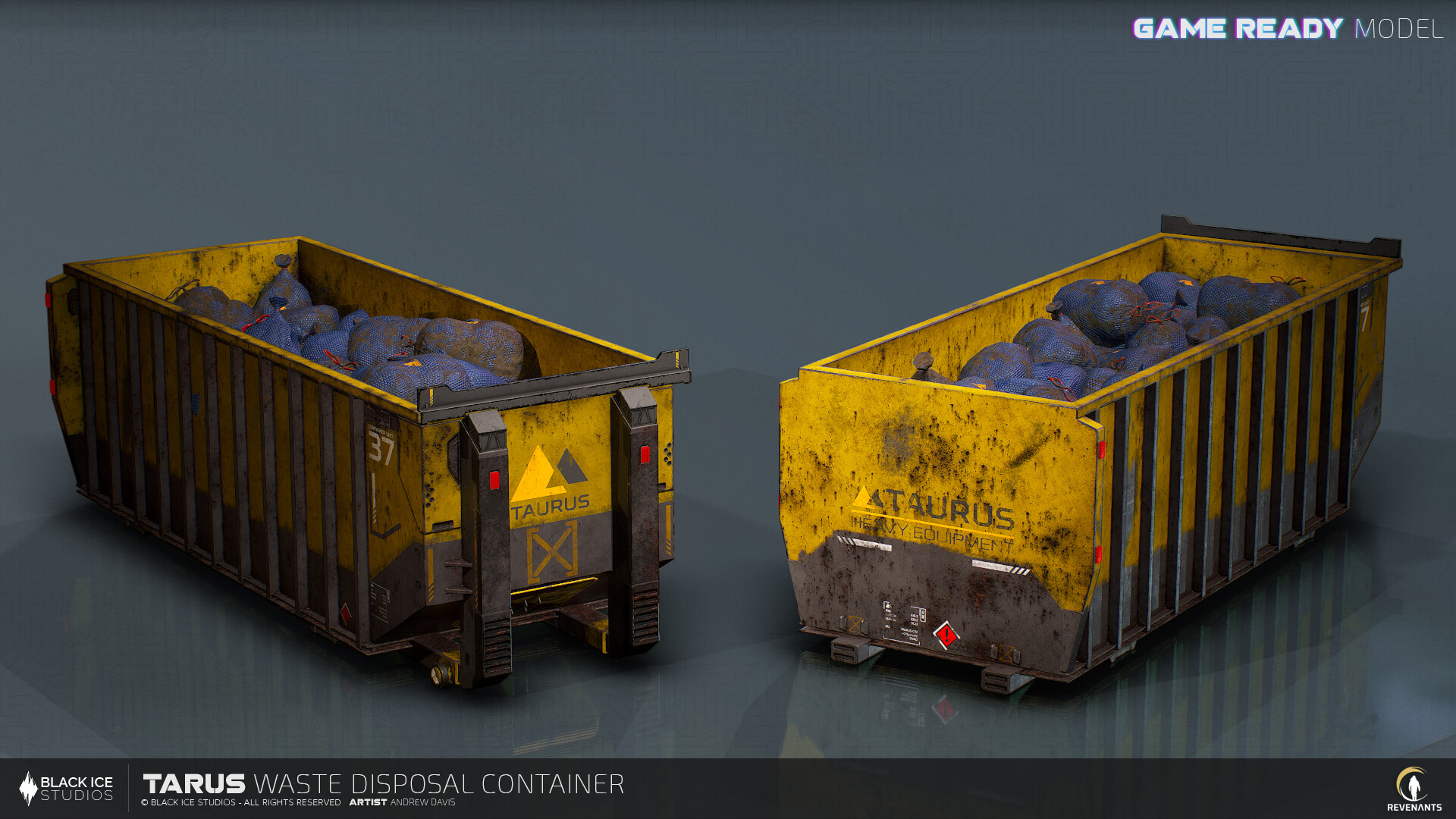The image displays a computer-generated model featuring two large, yellow waste disposal containers set against a dark gray background. Each container is adorned with gray patterns and contains numerous blue and black bags filled with waste. The text "Game Ready Model" is positioned in the top right corner, indicating the model’s suitability for gaming purposes. At the center of the image, the label "Terrace Waste Disposal Container" appears in white, followed by smaller, unreadable text. The containers, resembling industrial bins that would require a forklift or bulldozer for maneuvering, are reflected on the floor beneath them. Additionally, the bottom left corner displays the "Black Eye Studios" logo, while the bottom right shows the “Revenants” logo. The container on the left is marked with the name "Taurus" and features two vertical black columns likely designed for lifting the bin.